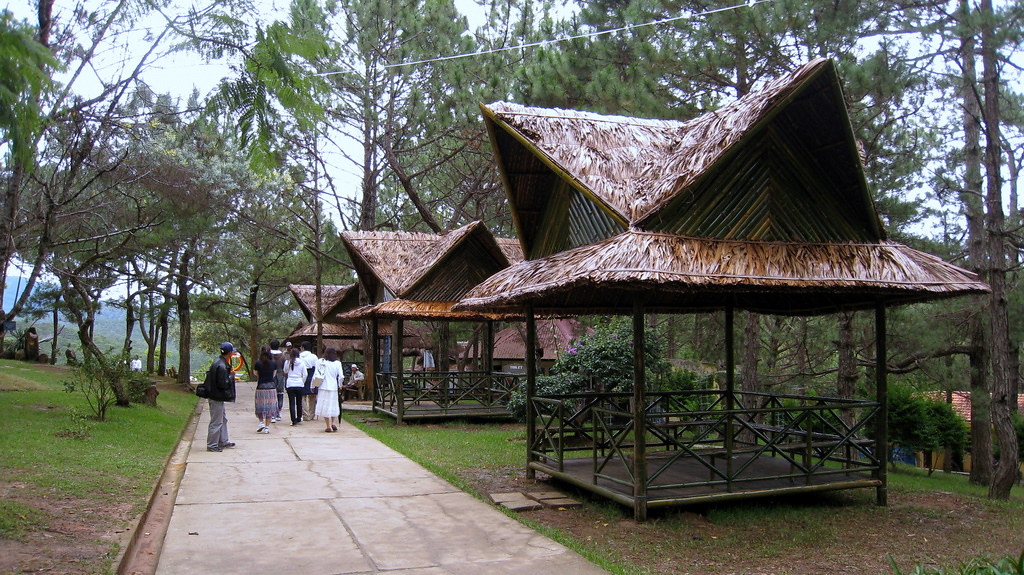The photograph captures a serene park, likely situated in East Asia, possibly Japan or China, characterized by a picturesque concrete walkway winding through a wooded landscape with the faint outline of mountains in the far distance. The focal point is a series of four pavilions adorned with intricate, thatched, straw-like roofs, each roof comprised of a lower tan-colored thatched section and an upper section forming four distinct peaks, resembling an origami star design when viewed from above. These structures, with a slight shine due to the lighting, house picnic tables and serve as quaint, open-air sitting areas. Scattered around the scene are various people; most notably, a man in a blue jacket with gray socks, wearing a baseball cap and carrying a bag, looks back toward a group of women, one in a white dress among them, while additional figures walk or sit along the sidewalk or further into the park. Overhead, electric power lines subtly cross the sky, adding a modern touch to the tranquil, natural setting.